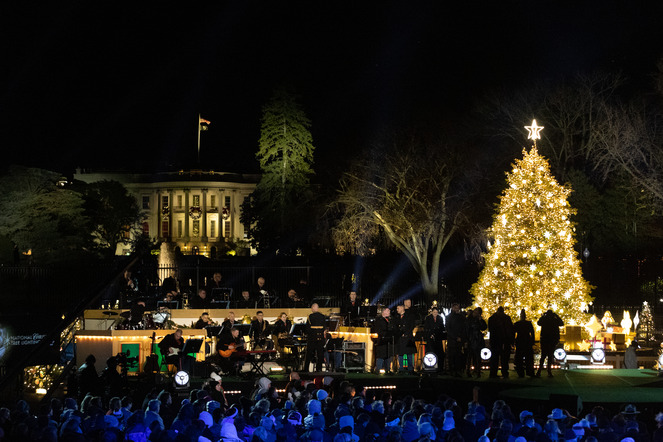The image captures an outdoor nighttime Christmas event set against the backdrop of a historically significant building, which appears to be the White House adorned with an American flag on top. The dark sky contrasts with the illuminated surroundings, including a grand, fully decorated Christmas tree to the right, glowing with golden lights and topped with a prominent star. The White House, positioned in the upper left of the image, is softly lit, with spotlit trees adding to the festive ambiance.

In the foreground, a stage is visible, occupied by an orchestra and several performers clad in formal black attire. Some performers are seated, likely playing instruments, while others stand, possibly singing. Beneath the stage, an audience is gathered, seated and bathed in a bluish glow. The scene is vibrant with warm lighting, emphasizing the holiday celebration, likely a Christmas tree lighting ceremony, underscored by the distant, elegant lighting of the White House and surrounding trees.